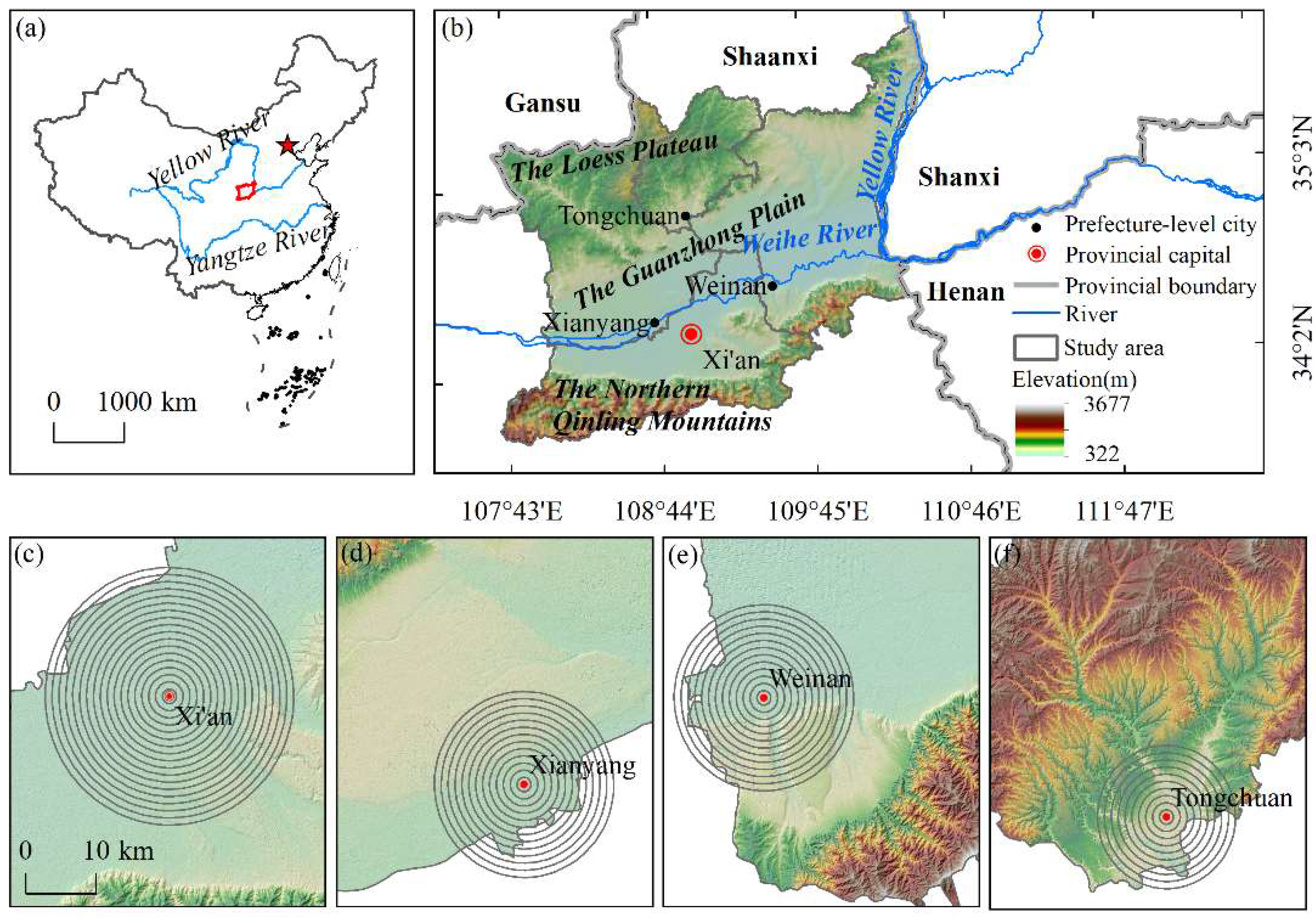The image displays six maps of various Chinese regions, labeled from A to F. Map A, situated at the top left, includes labels for the Yellow River and the Yangtze River. Map B offers a detailed topographic view, highlighting areas such as Gansu, Shaanxi, Henan, the Guangzhong Plain, the Northern Qinling Mountains, and other significant texts. These regions are depicted in green and brown, with rivers shown in blue. Below Map B, there are four smaller maps labeled C, D, E, and F. Each of these highlights specific cities—Xi'an, Xianyang, Huainan, and Tongchuan — with concentric rings around each urban area, suggesting focused zones, though without an explicative legend. The overall presentation accentuates the provincial capitals, borders, valleys, and mountain ranges across China, blending vibrant colors for clear geographic and topographic differentiation.